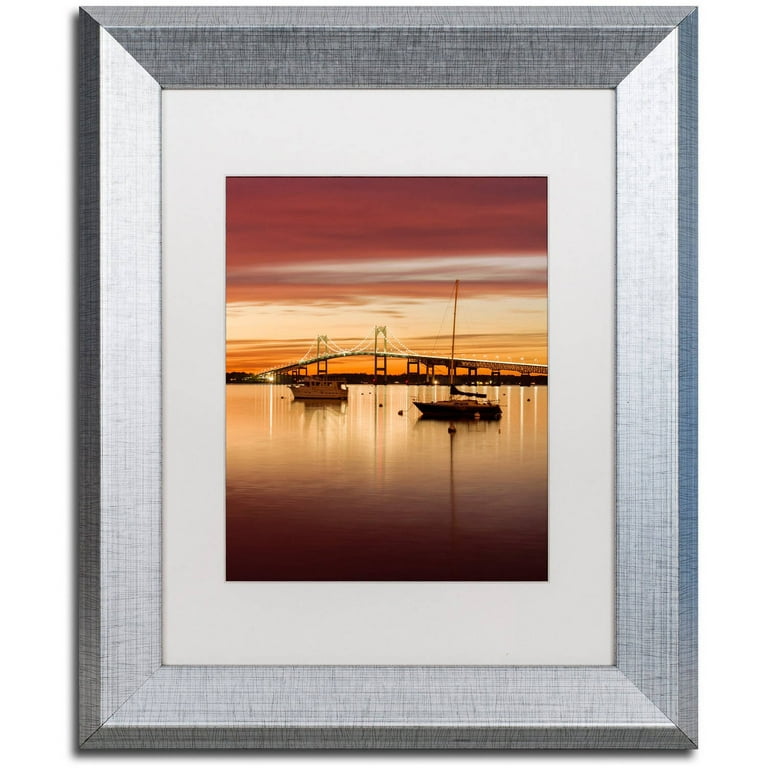A framed photo captures a serene sunset scene featuring a lake with two boats in front of an illuminated bridge. The frame is large and metallic, with a white border surrounding the image. The boat on the right is black and appears closer, featuring a tall pole with a flag, while the boat on the left is smaller and white. Buoys surround the boats, adding to the tranquil setting. Above the bridge, wispy gray clouds thicken towards the top, and the sky exhibits a reddish-purple and orange hue. The water beneath the boats appears darker in the foreground and lighter near the horizon due to the sun's reflection, enhancing the peacefulness of the evening scene.